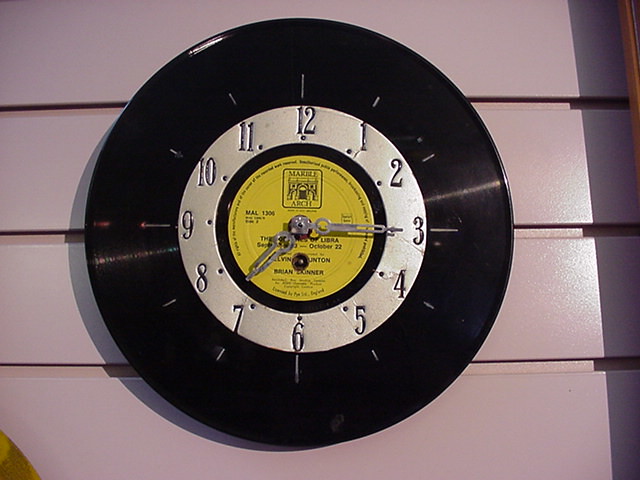The vibrant image showcases a medium purple wall made of slatted paneling, with evenly spaced grooves between each board that are also painted purple. Mounted on the wall is a distinctive clock, designed to resemble a vintage vinyl record. The clock features a thick black border, reminiscent of an album's outer edge, and a silver inner circle marked with black numbers indicating the hours. The center of the clock is highlighted by a yellow circle with indecipherable text, adding to its retro charm. The sleek silver hour and minute hands further enhance the illusion of an old-fashioned record.